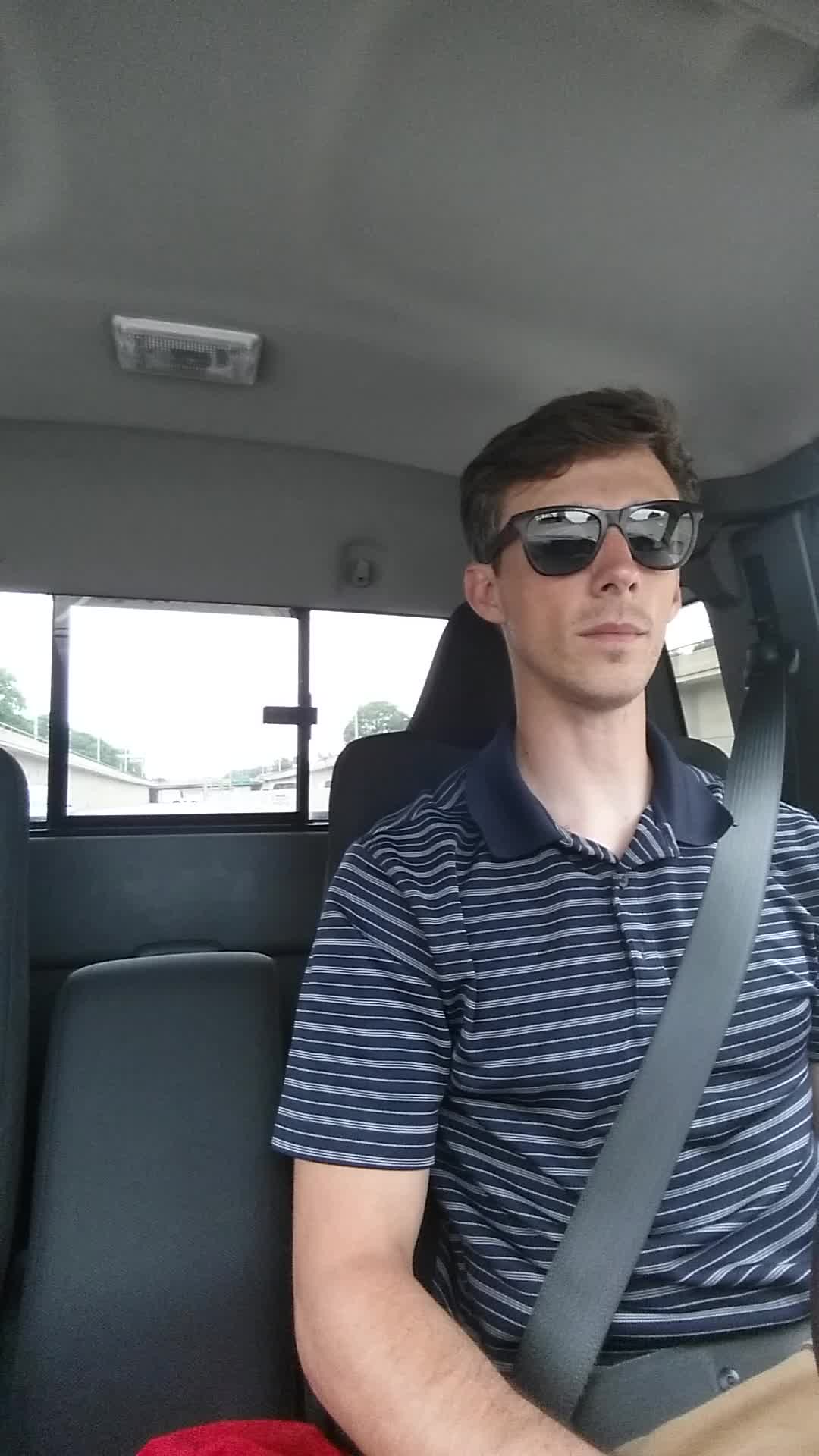This vertical rectangular photograph captures a man sitting in what appears to be a truck with a gray interior. The man, with short brown hair combed to the side and a mustache, is wearing dark sunglasses and a navy blue collared short-sleeved striped polo shirt. The shirt features navy blue and lighter gray horizontal stripes extending from the collar down to the sleeves. He is securely fastened with a grayish seat belt across his chest and waist and is possibly wearing khaki pants, although this detail is mostly obscured.

The driver, presumed to be the man in the photo, is seated in the middle seat with his left arm visibly extended forward. In the vehicle's interior, the back windshield features three nearly square windows with the full center window and partial views of the left, right, and side ones. Notably, the center window includes a smaller sliding section. Above him on the ceiling, there is a switch or box, likely a light fixture. A gray armrest is positioned in the middle, pushed up, revealing a red object, possibly a hat, near his left elbow and the seat. The photograph was taken during daylight, and the overall setting appears bright, as indicated by the white light visible through the windows behind him.